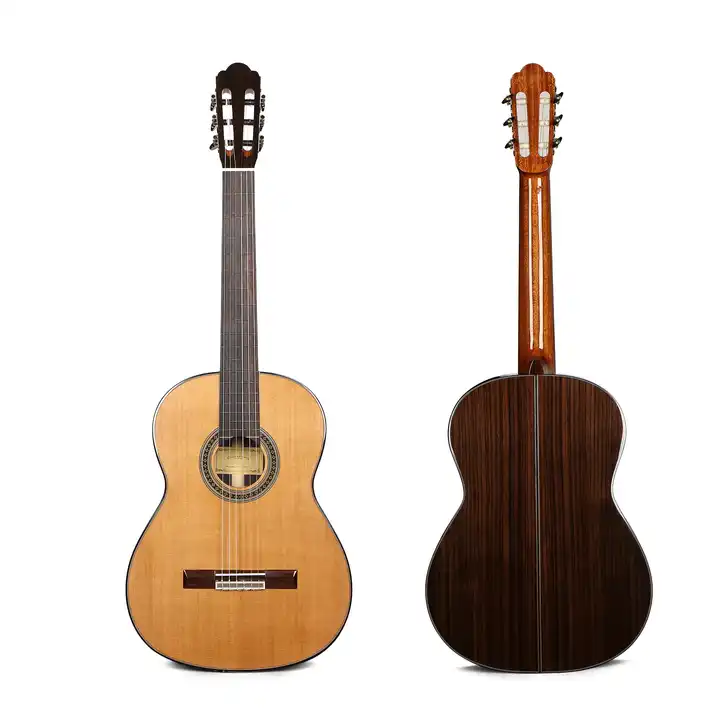The image features a classical guitar depicted through two side-by-side pictures, showcasing both the front and back views. The guitar in the left image stands straight up with its base on the ground and its neck extending towards the top of the frame. The front of the guitar has a traditional light brown color with a gray neck featuring slender white strings. A dark brown pegboard with silver tuning knobs is located at the top of the neck. Below the neck, the guitar’s body is light brown with a dark brown border. There is a circular sound hole with a black border beneath the neck, and a dark brown rectangular piece of wood horizontally attached near the bottom of the guitar where the strings are secured.

The right image shows the guitar's back, which is a very dark brown, contrasting with the lighter shades of the front. The back of the neck and the pegboard are darker brown compared to the light brown of the front neck. The overall appearance of the guitar suggests that it is relatively new and likely intended for beginners. There is no visible text on the guitar that can be easily read in the picture.